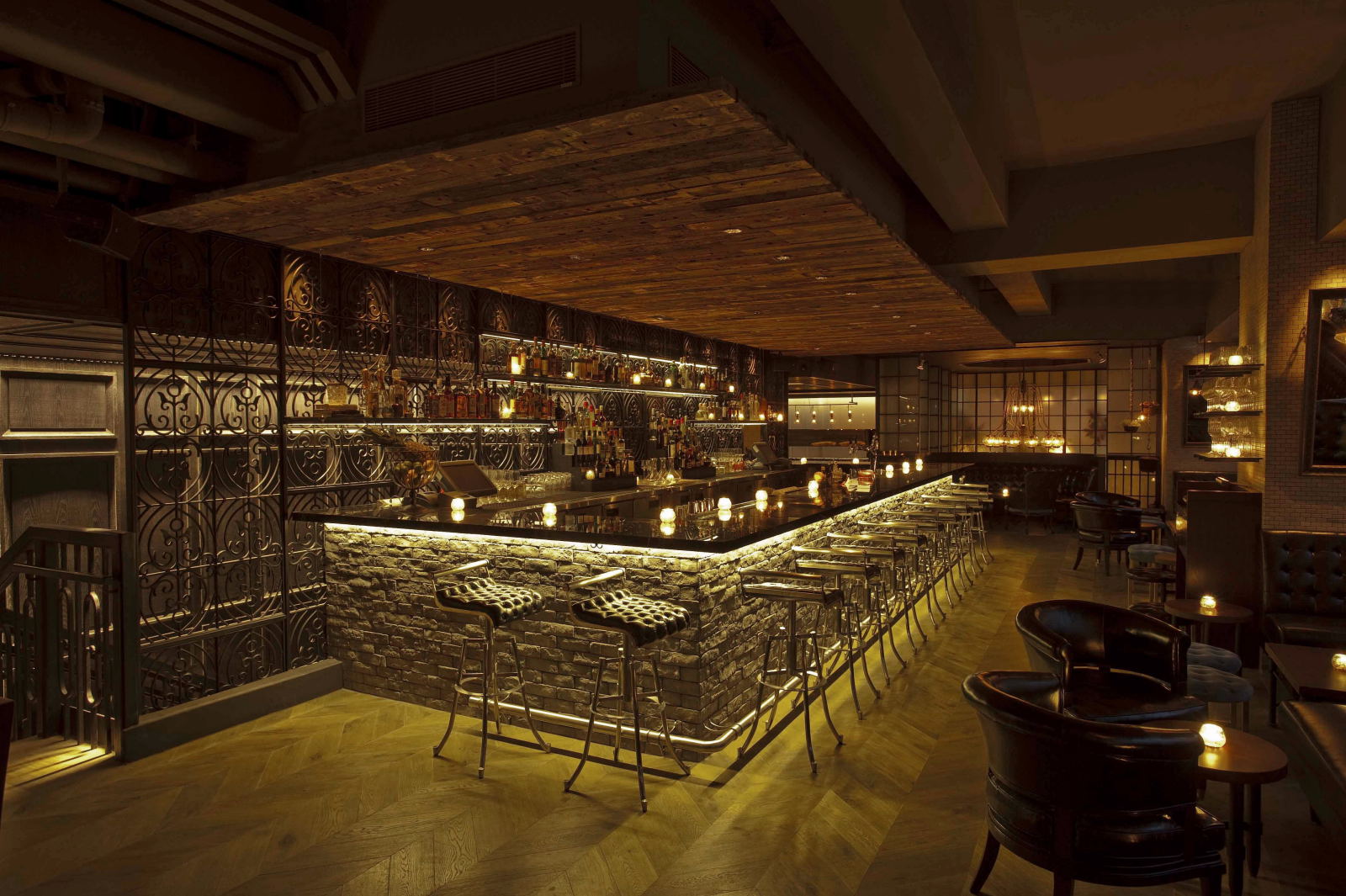This image depicts a romantic and dimly lit, upscale bar with a sophisticated aesthetic. The bar has a distinctive L-shaped design with a reflective black bar top and a grey stone siding. Along the bar are backless, or nearly backless, stools with puffy black padding, lending an air of exclusivity. The bar features under-lighting and a metal footrest for added comfort. Tiny candles in glass orbs illuminate the space, placed both on the bar and on the small circular tables at nearby booths. These booths are adorned with leather chairs and benches, offering cozy seating arrangements. In the background, checkered Japanese-style windows add a cultural touch, while the ceiling above the bar has a reclaimed wood appearance with exposed ventilation and black metal detailing, enhancing the industrial-chic vibe. A staircase begins on the very far left, subtly indicating another level or area. The atmosphere is complemented by herringbone light wood flooring and dim lighting that enhances the romantic and intimate setting. Additionally, a POS system is visible behind the bar, signifying the bar's operational setup. The sophisticated details and meticulous design elements suggest that the image might be slightly AI-generated.